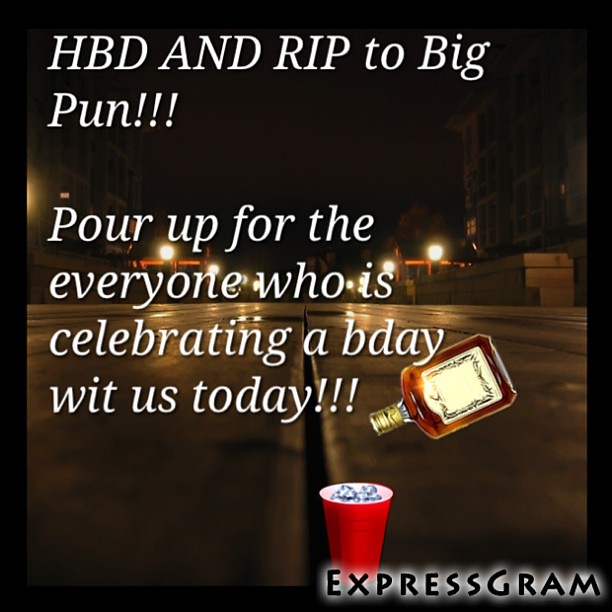The image is a graphic design featuring a nighttime urban scene with a cracked cement street in the foreground, viewed from a low angle. The background reveals some distant buildings and street lights, under a dark night sky. Superimposed over the photograph, from top to bottom, is the text: "HBD and RIP to Big Pun!!!" followed by "Pour up for everyone who is celebrating a bee day with us today!!!". The text overlays are accompanied by a crudely cropped image of a tilted Hennessy bottle pouring into a red plastic cup filled with ice. The bottom right of the image is marked with the word "Expressgram" in black text, surrounded by a smoky white border. Overall, the scene portrays a somber yet celebratory mood, blending urban grit with elements of festivity.